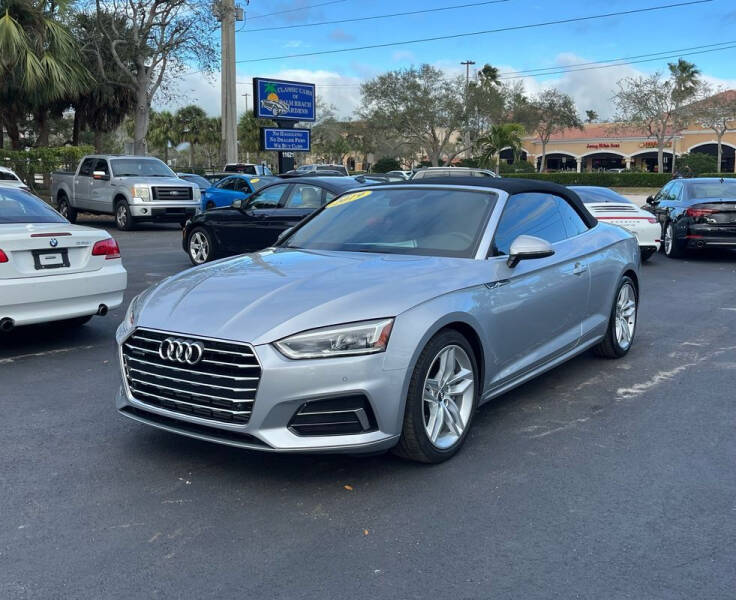The image captures a sleek, silver-grey Audi A5 Roadster convertible, prominently featured in a bustling parking lot. The Audi, adorned with its iconic four-ring logo on the grille and sporting a dark-colored cloth soft top, exudes a refined and aggressive aesthetic with its large metallic grill and slanted headlights. Positioned at an angle towards the left, this two-seater convertible stands out amidst an array of vehicles. Behind the Audi, a variety of sports cars, including BMWs and Porsches, are visible, many bearing yellow stickers on their windshields, signifying a possible used car lot. The parking lot is paved with dark gray asphalt and populated with additional cars and trucks. In the background, a blend of commercial buildings, likely a strip mall with blue signs, stretches across the scene under a sky mottled with white clouds. Power lines and light posts are visible, framing the area along with some greenery and trees, adding depth to the daytime setting.